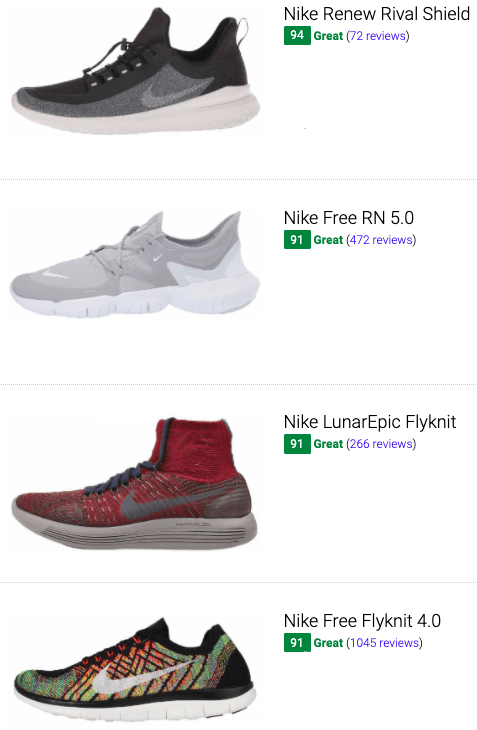This image is a sleek advertisement for Nike sneakers that you might see online. The background is pure white, providing a clean and minimalist canvas to highlight the product. Four sneakers are vertically aligned in a single column, each separated by a light gray line. All the sneakers are showcased in a profile view, facing left.

At the top, the first sneaker is a blend of black and gray with a small Nike swoosh. It features a white sole, and next to it, text reads "Nike Renew Rival Shield." A green box states "94 Great," which appears to be a rating, with "72 reviews" noted in parentheses.

The second sneaker is predominantly gray with a white bottom and a Nike swoosh. Accompanying this image is the label "Nike Free RN 5.0." Beside it, the green rating box indicates "91 Great," followed by "472 reviews" in parentheses.

The third sneaker in the sequence has a stylish mix of red and gray, with a gray swoosh and white sole. The design rises higher up the ankle, resembling a high-top sneaker. The red upper part contrasts with the rest of the shoe, labeled as "Nike LunarEpic Flyknit." The green box specifies a "91 Great" rating, with "266 reviews" in parentheses.

At the bottom, the fourth sneaker boasts a colorful combination of green, orange, and black, enhanced by orange and black stripes. It also has a white swoosh and white sole. The adjacent text identifies it as "Nike Free Flyknit 4.0," with a rating of "91 Great" in the green box and "1045 reviews" noted in parentheses.